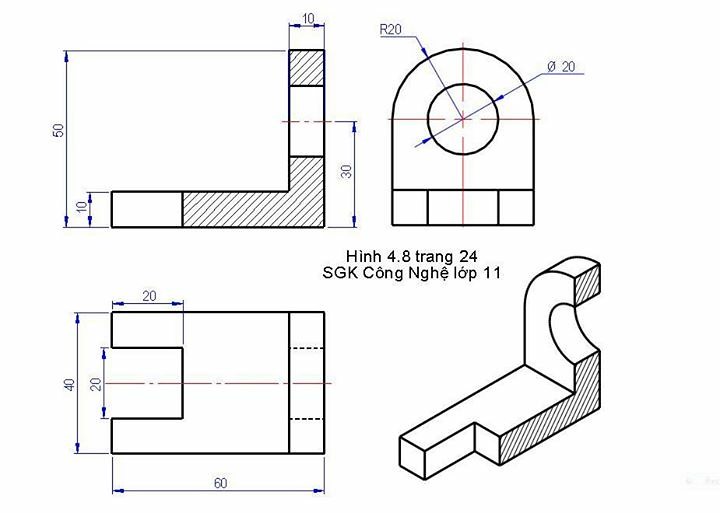This image is a detailed black-and-white schematic diagram on a white background, depicting various shapes and dimensions, likely used for a manufacturing or assembly process. The visual includes four main geometrical shapes, each annotated with specific measurements.

In the top left corner, there is an L-shaped figure, rotated 180 degrees counterclockwise. The bottom part of this L-shape is labeled with a length of 50 units, although the units are unspecified. The height of the left side of this L is marked as 10 units, with lines and arrows indicating these dimensions. 

The bottom-left section of the image contains a rectangle with a square cutout in its middle-left side. The bottom edge of the rectangle measures 60 units in length. Additional dimensions are noted with arrows, such as a height of 40 units along the left side and a top segment measuring 20 units.

In the top right corner, there's an arched shape featuring a central circle marked with an R20, indicating its radius. This shape has text beneath it that reads: "HINH 4.8 TRANG 24" followed by "SGK KONG NGHE LOP 11," which appears to be in Vietnamese.

Finally, the lower right corner features another shape, somewhat three-dimensional with parts shaded in using diagonal lines. This shape, unlike the others, lacks clear labeling but contributes to the overall technical appearance of the diagram.

The entirety of the image is drawn with simple black lines against a stark white background, resembling a page from a technical manual or a set of assembly instructions.